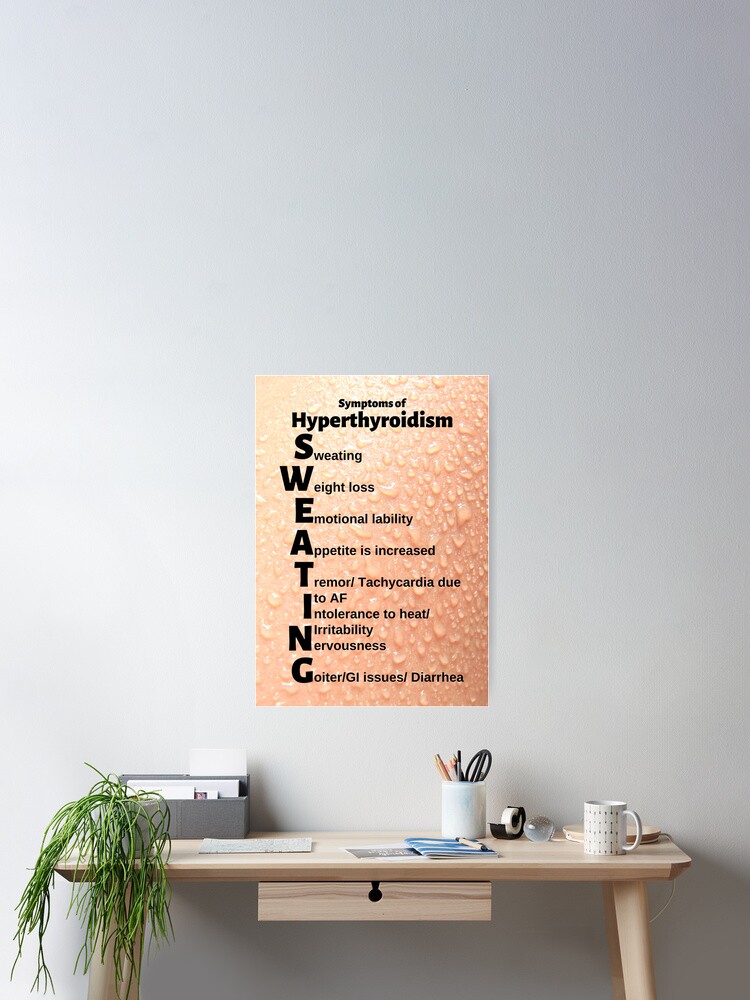The image depicts a small, natural wood desk positioned against a vast white-to-gray gradient wall, with light coming from the left and the desk slightly off-center to the right in the lower portion of the frame. The desk, which is rectangular and supported by four legs, features a single drawer with a dark-colored knob. Resting on the desk are various items: a white, adjustable desk lamp placed at the back right corner; a white coffee mug in front of the lamp; a white jar containing pens, pencils, and scissors; a black tape dispenser with clear tape; and several papers, notebooks, and notepads scattered around. Additionally, there is a sad-looking, drooping small potted plant in front of a metal box filled with papers. Mounted on the wall above the desk is a poster, primarily orange with water droplets, possibly resembling skin, that reads "Symptoms of Hyperthyroidism" with the word "sweating" vertically aligned and accompanied by unreadable details for each letter. The stark contrast of the minimalistic workspace against the vast wall emphasizes the compact nature of the desk area.